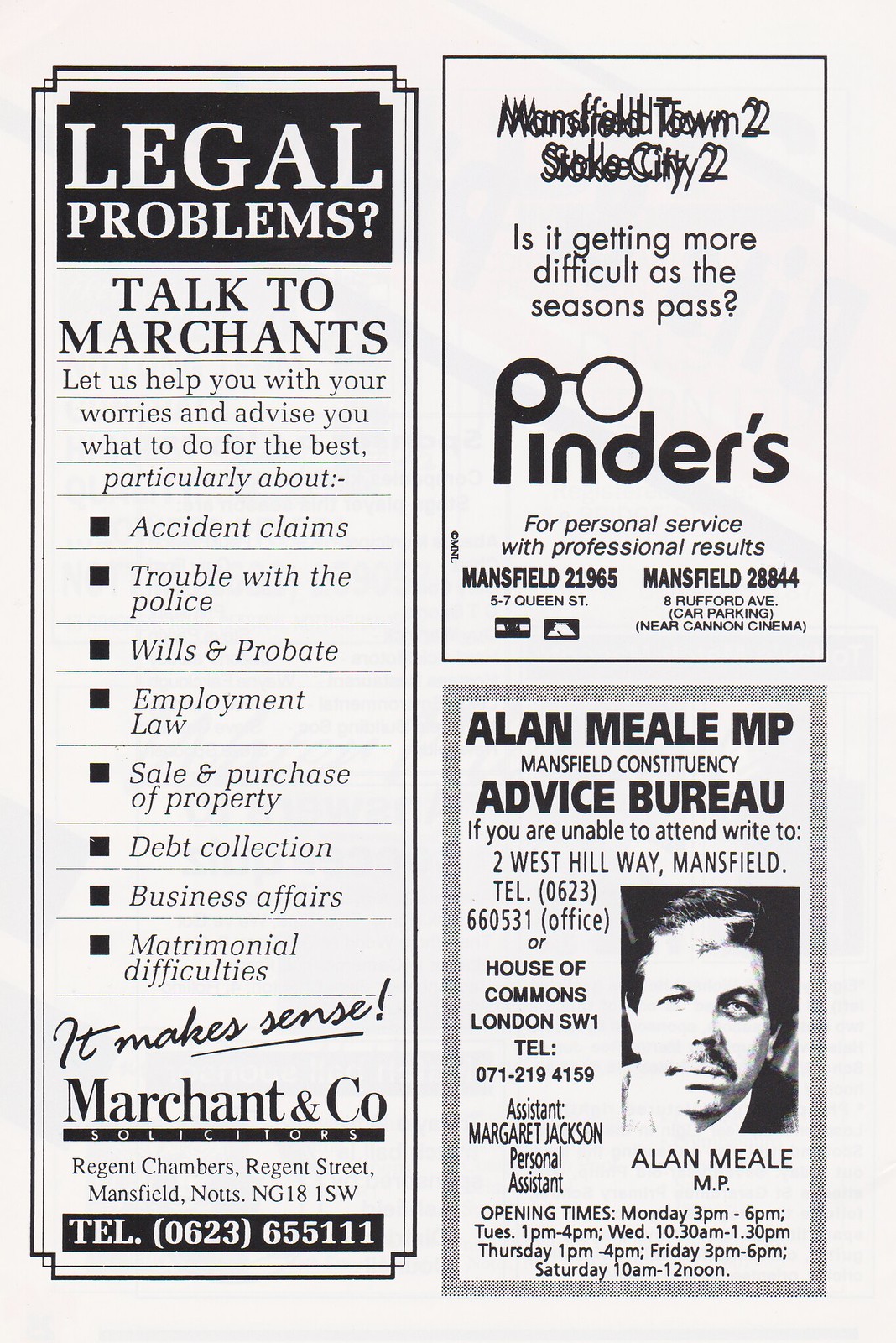The image is a sectioned advertisement poster displaying three distinct ads. The first ad, a long rectangle on the left, starts with "LEGAL PROBLEMS?" in bold, white text on a black background. It invites potential clients to "Talk to Merchants" and promises to help with various issues, listing accident claims, troubles with the police, wills and probate, employment law, sale and purchase of property, debt collection, business affairs, and matrimonial difficulties. The ad concludes with "It makes sense!" and provides contact information for Merchant and Co., Solicitors at Regent Chambers, Regent Street, Mansfield, NOTTS, NG18 1SW, alongside the phone number (0623) 655111.

The second ad, situated to the right, is for an eyewear service. It features the blurry text "Mansfield Town 2, Stokes City 2" followed by a cryptic question, "Is it getting more difficult as the seasons pass?" The ad depicts eyeglasses forming the letter "P" and introduces "Pinders" with the tagline "Personal service with professional results." Contact details include Mansfield 219655, 27 Queen Street, and Mansfield 28844 with additional location information near Cannon Cinema at 8 Rufford Avenue.

The third ad promotes Allan Meale MP's Mansfield Constituency Advice Bureau, providing guidance to constituents. It lists an accessible address and contact details, suggesting individuals write to a specific address at the House of Commons in London if unable to attend in person.